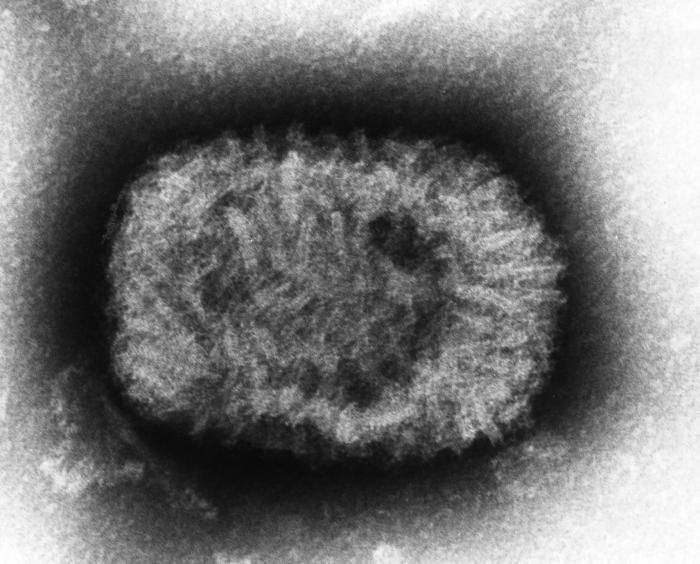This detailed black-and-white image appears to be taken by a machine designed to view specific layers of a subject, possibly resembling an x-ray or ultrasound. The image features a broad, whitish periphery that transitions into a dark ring or circle toward the center. This dark ring, reminiscent of a black hole, encloses a cluster of elongated, worm-like shapes. These shapes are densely packed together, forming an intricate mishmash primarily in the middle of the circle, layering haphazardly upon one another. The overall texture is very grainy and spotty, with the graininess persisting throughout but fading into white light at the edges. The elongated shapes create a sense of chaotic organization, with long ovals pointing inward and intertwining to create an almost ring-like structure around the center.